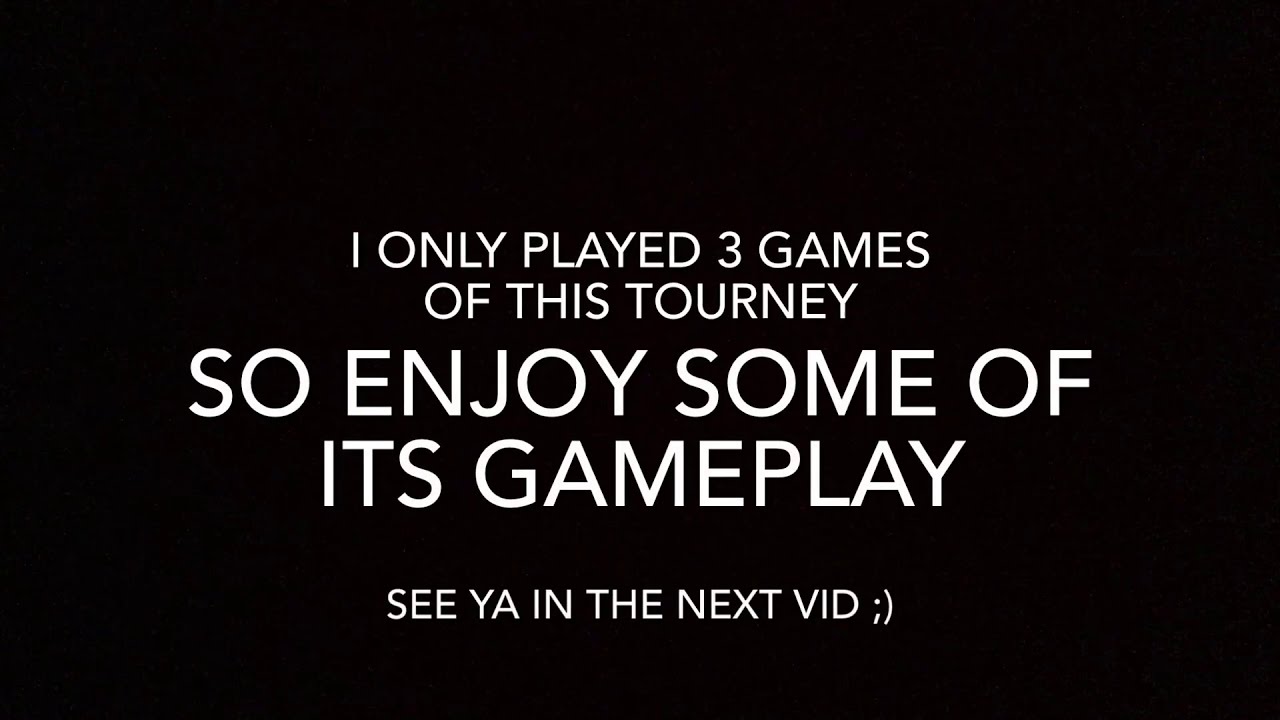Against a black background, centered slightly below the middle, is a series of white, uppercase text lines in a very straight, bold font. The top two lines read, "I ONLY PLAYED THREE GAMES," followed by "OF THIS TOURNEY." In larger font, the next line states, "SO ENJOY SOME OF," followed by "ITS GAMEPLAY." Lower down, the smallest text says, "SEE YA IN THE NEXT VID," followed by a semi-colon and a closed parenthesis, resembling a winking emoticon. The visually striking design seems apt for an end frame of a video game highlight reel.